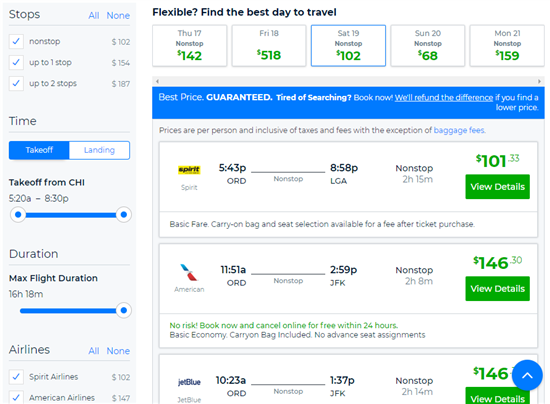The image captures a screenshot of a comprehensive flight search and booking website, showcasing a well-organized interface designed to streamline the travel planning process.

On the left side of the screen, a prominent column approximately taking up the left quarter of the page features various filter options to refine the flight search results. At the top of this filter column, the heading "Stops" is displayed in bold black font. Directly to the right of this heading, the options to select "All" or "None" are available. Below this, users can filter by the number of stops, with options for "Non-stop", "Up to 1 Stop", and "Up to 2 Stops", each accompanied by respective price ranges for convenience. Further down, the column provides filters for takeoff and landing times, allowing users to input their preferred departure times from the CHI airport specifically. Following this, a slider is available for setting the desired flight duration, enabling users to see results that match their time preferences. Additionally, there is an airline filter to narrow down choices based on preferred carriers.

On the right side of the screen, the interface's top section highlights the "Flexible" option, encouraging users to find the best day to travel. Directly beneath this, the interface presents several selectable dates with their corresponding pricing options. In this screenshot, the "Saturday 19th Non-stop" option, priced at $102, is highlighted with a blue border indicating its selection. 

Below this date selection, the website displays the flight listings and their pricing for the selected day. Available flight results include options from Spirit, American, and JetBlue Airlines, providing users with a range of choices depending on their airline preference and budget constraints.